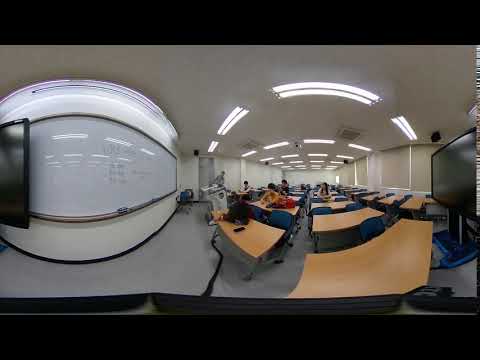The image depicts a fisheye view of a college classroom. The room is furnished with numerous brown wooden tables, each accompanied by blue chairs neatly tucked in. Several tables, approximately four or five, are occupied by students. The walls are white and adorned with a large whiteboard on the left side, featuring some handwritten notes. A small blackboard is visible as well. Fluorescent tube lights are installed on the ceiling, illuminating the gray floor below. The central area of the image is slightly distorted due to the fisheye effect, creating a circular, fishbowl appearance. An instructor stands near the whiteboard, though the details of their attire are unclear. Additionally, a television or some kind of monitor is placed on the right side of the room, presumably for educational use. Among the students, one individual in the center stands out, wearing a yellow shirt and holding a red backpack.